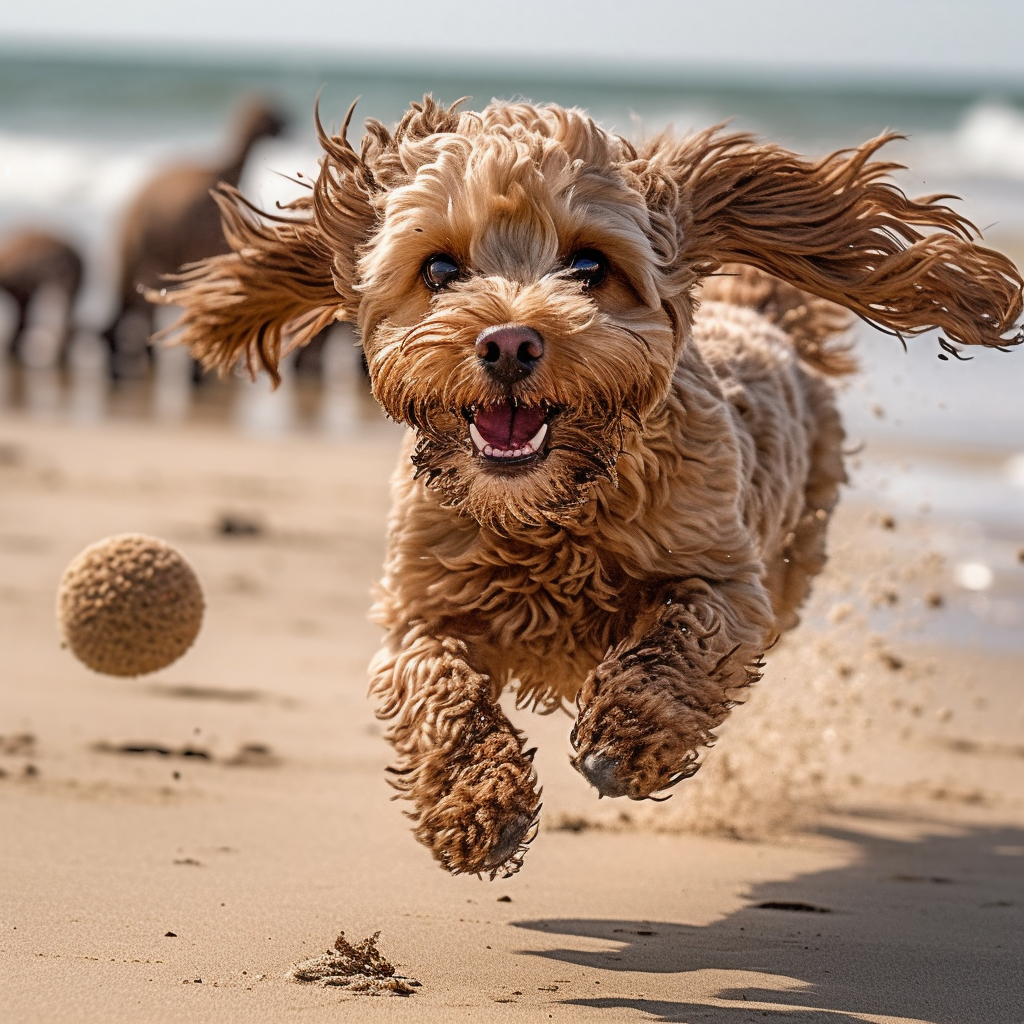In this captivating close-up image, a small Yorkie-like dog is joyfully running on a sandy beach towards the camera, creating an almost lifelike feel. The endearing pup, likely less than a foot tall with curly and wavy fur in shades of brown and beige, has its ears flopping in the wind and its mouth open, exuding excitement. Bright brown eyes add a touch of liveliness, and its fur appears wet and sandy. The dog is airborne, kicking up sand underneath and leaving a trail of sandy paw prints behind. Next to the dog, a small brown ball floats, suggesting it was being chased. Despite the focus on the dog, the background reveals a gray, muted sky and bits of water, with indistinct, brownish animals that could be more dogs or horses. The horizon of the ocean is faintly visible at the top, while blurred images of birds add to the beach setting, enhancing the scene's dynamic and cheerful atmosphere.